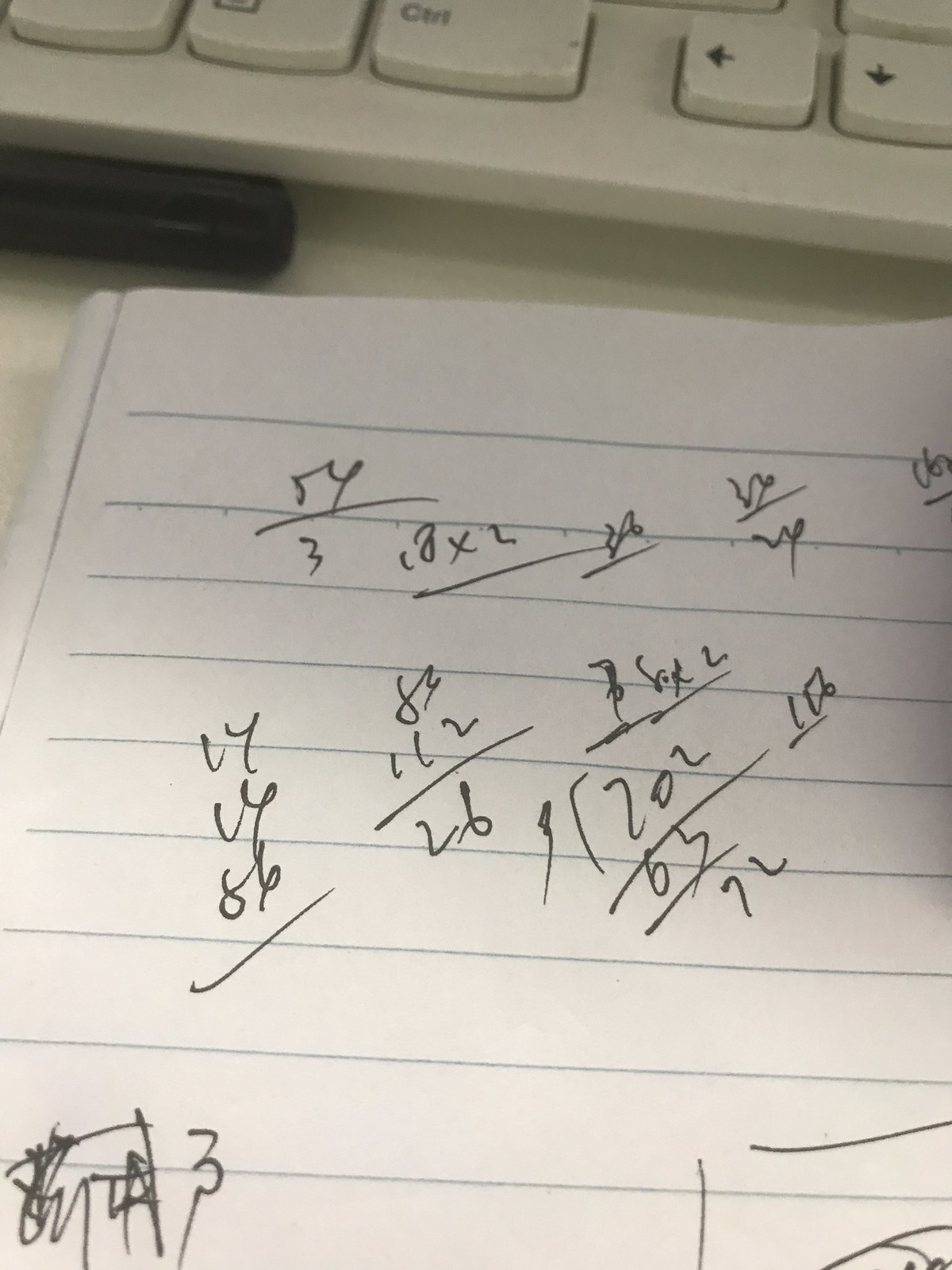This image captures a cluttered scene of handwritten arithmetic and doodles on a sheet of lined paper positioned below a slightly soiled computer keyboard. The upper left and central sections of the paper feature various mathematical operations executed in pen, including addition, multiplication, and number listings. Notable figures such as "54/3," "18x2," and "26" with a horizontal line beneath are visible, alongside scattered totals like "86," "83," and "112/26." Incomplete and struck-out equations, like a "3" with an extended tail, add to the chaotic nature of the working area. The lower right corner of the paper reveals random lines and stray marks suggestive of idle doodling. The entire setting conveys an atmosphere of concentrated problem-solving amidst a somewhat disorganized workspace.